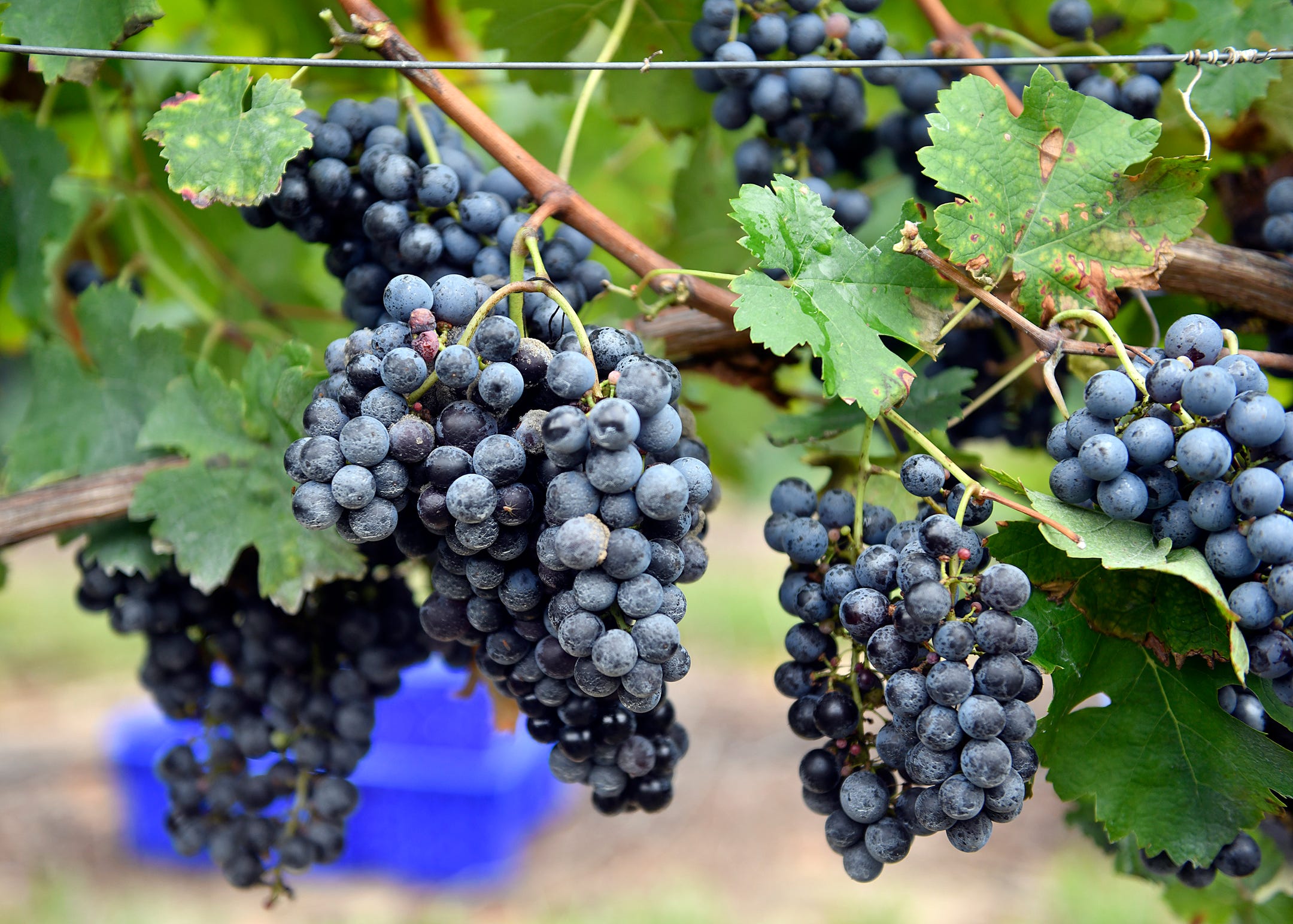This photo captures a close-up view of an outdoor grapevine densely adorned with multiple clusters of dark blue, almost black grapes. The fruit, spherical in shape with a slight purplish tint and a whitish bloom on some, hangs prominently from the brown vines amidst lush, dark green leaves, some of which show signs of browning. The scene includes a total of seven visible clusters of grapes – three in the foreground and four more in the background, with two partially visible. Overhead, a black rope stretches across the top of the image, likely providing support for the vine. Additionally, a blurred, blue box-like structure is faintly visible on the left side of the image, adding depth to the composition.